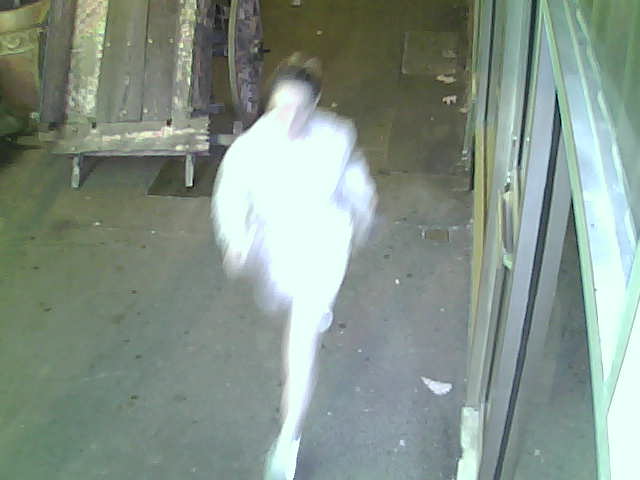This photograph, likely a screenshot from a high-mounted security camera positioned at least one story up, captures a dynamic outdoor scene. At the center of the frame, a woman dressed entirely in white is caught mid-step, walking past. Her attire includes a white sweater, white shorts, and running shoes. Despite her motion making her silhouette slightly blurry, details such as her blonde or light-colored hair styled in a bun are discernible. To the right side of the image, a metal door frame intrudes into the frame, providing contextual depth. Behind the woman, a large dumpster and possibly a wooden object are visible, further enhancing the setting. The ground beneath is a mix of cement and tiles, solidifying the impression of an outdoor environment. The clear background contrasts with the woman's movement, highlighting her as the focus of this momentary capture.